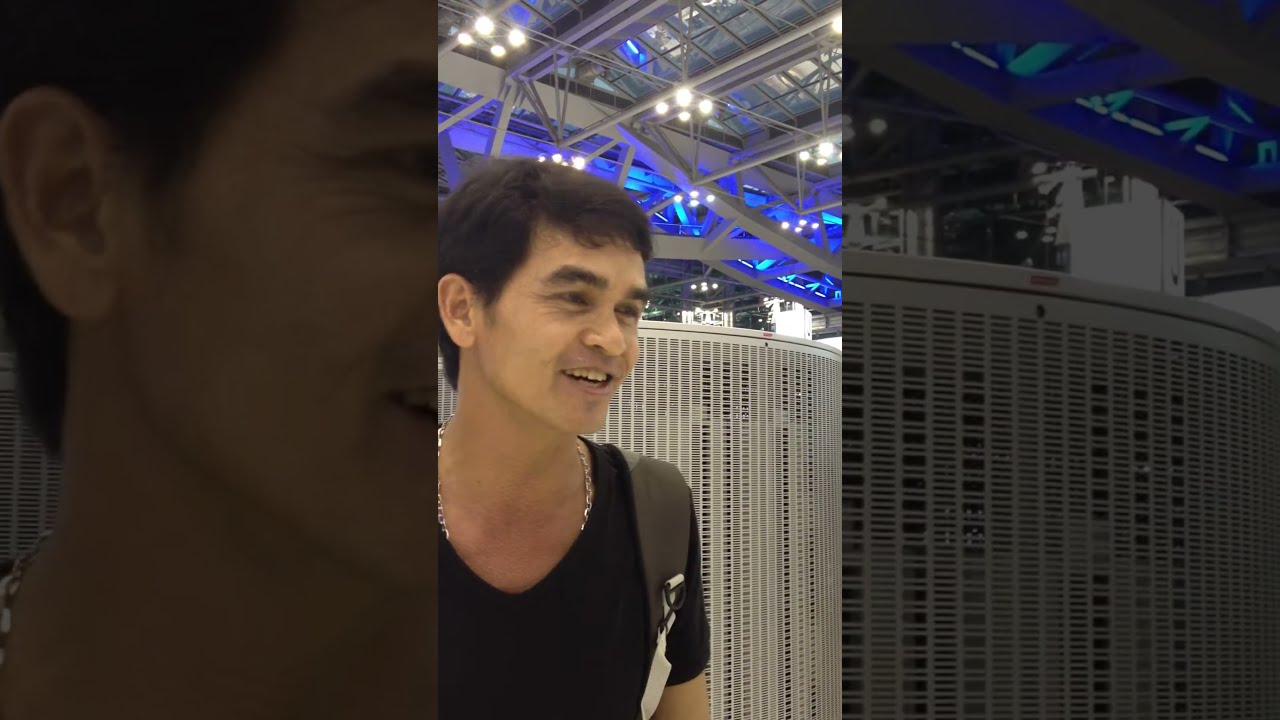This detailed image captures a serious-looking man with a darker complexion, short black hair, and brown eyes, centered in the frame. He is gazing off to the right. He is adorned in a black and gray outfit composed of a jacket or sweater over an undershirt, with two visible straps and a metal chain necklace. The indoor setting features a ceiling crisscrossed with beams, illuminated by numerous lights, many of which cast a blue hue across the scene. Behind him are large structures that resemble fans and possibly windows, hinting at daylight streaming in. The overall color palette includes shades of gray, black, silver, blue, tan, and white. The composition's focus is the man's face and upper torso, leaving his exact activity and environment somewhat ambiguous, although it hints at a large, industrial-like building.